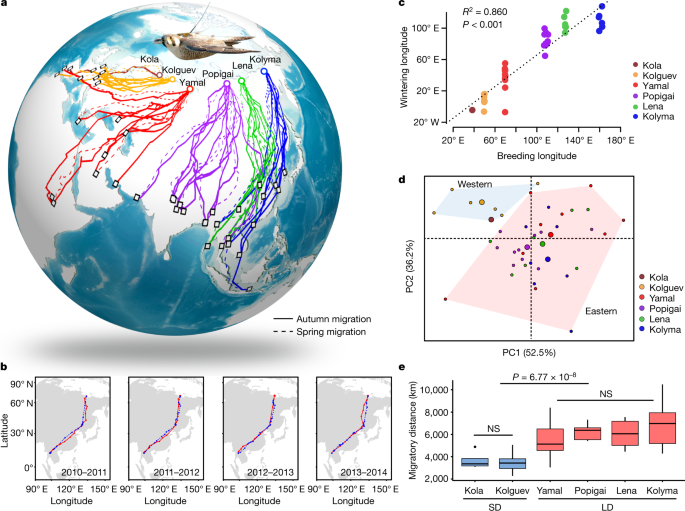The image showcases a highly-detailed scientific diagram centered around the migratory patterns of a bird, possibly a species native to the Northern regions. The diagram features a globe focusing on parts of Asia, Europe, and Northern Africa, with various colored lines representing the bird's flight paths. The paths span from the frigid northern regions of Russia, through Europe, and down towards Africa and the Pacific, even nearing Australia.

A visual depiction of the bird, which is white, gray, and brown, is situated atop the globe, connected via a long black line, possibly indicating a tracking device. Accompanying the globe are several graphs and scatter charts, elucidating specific migratory details such as “breeding longitude” and “wintering longitude,” arranged on different axes. The data is dense and covers both the autumn and spring migration periods.

Additionally, there's a series of smaller maps beneath the main globe image, each representing the bird's migration routes for different years, specifically from 2010 to 2014. Locations mentioned within the image include Kola, Kolgev, Yamal, Popigai, Lena, and Kolyma, highlighting key regions in the bird’s migratory journey. The rich amalgamation of graphical elements and data points provides a comprehensive overview of the bird's migration patterns and related scientific insights.